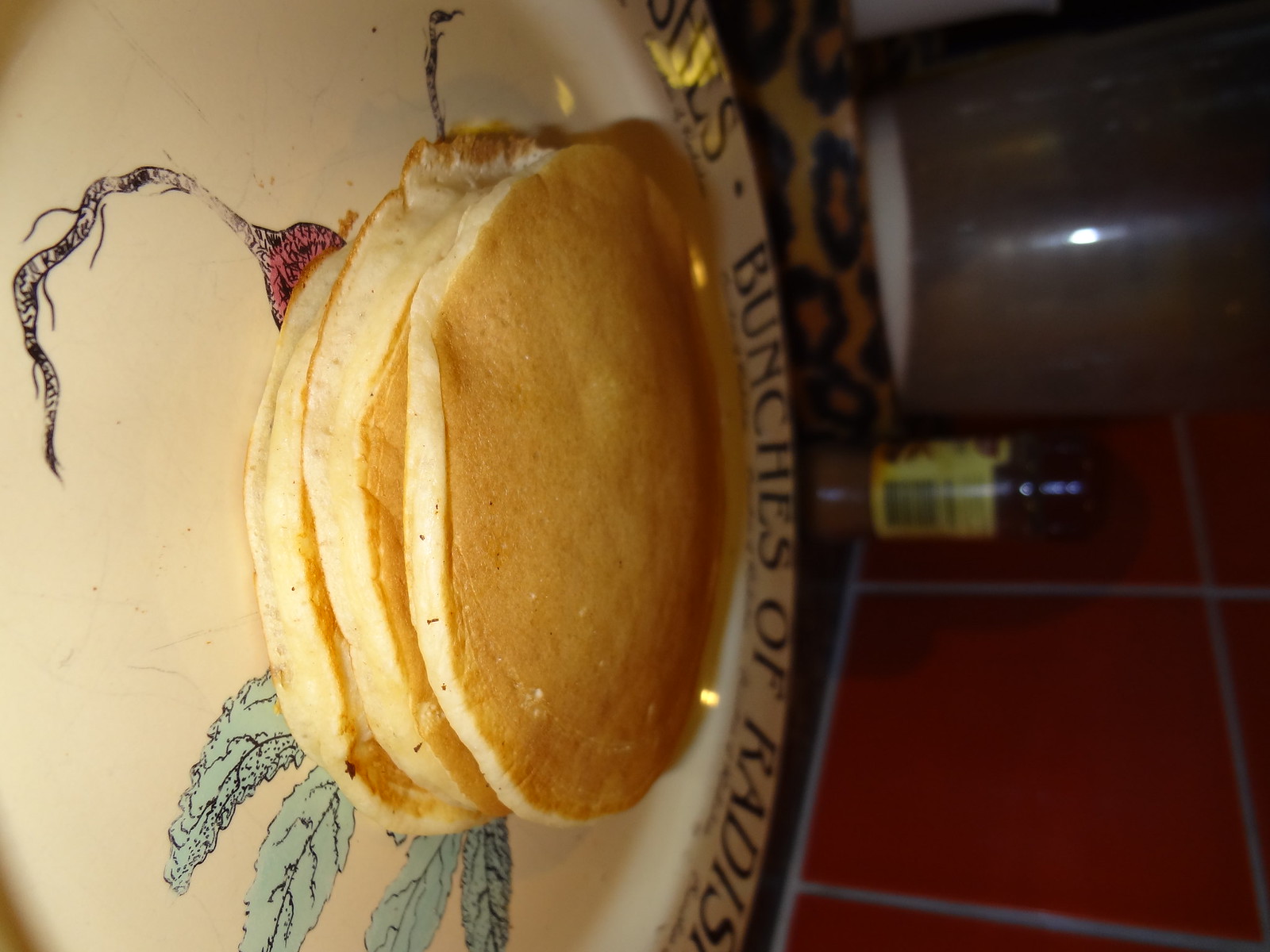The image is a detailed, color photograph taken inside a dimly lit restaurant, oriented incorrectly at a 90-degree angle. It features a close-up of a plate with three medium-sized, light brown pancakes with white edges stacked in the center. The plate is adorned with an illustration of radishes, positioned underneath the stack, and bordered with repeated text that reads "Bunches of Radishes" in black letters around its rim. In the background, there is a square-patterned, red-tiled wall with gray grout, contributing to the overall dark ambiance. Additionally, a bottle or spice container with an unreadable label can be seen, adding to the background details.